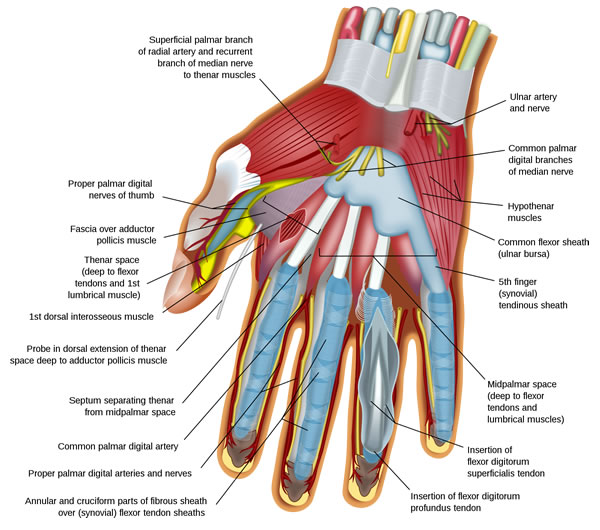This is a meticulously detailed, computer-generated anatomical illustration of a human hand, reminiscent of the diagrams one might encounter in an educational setting. The image showcases the intricate structure of nerves, muscles, tendons, and bones within the hand, beginning from the wrist at the top. Vertical lines, resembling tiny tubes, are color-coded in red, green, and yellow to differentiate between various anatomical elements. Accompanying the hand are labels with small black text connected by lines to specific features, aiding in identification. For instance, one label identifies the "common palmar digital artery," with an arrow pointing precisely to its location. The muscles are depicted in red, providing a stark contrast against the blues and grays representing other tissues. The bones stand out in white, completing this comprehensive visual guide to the hand's internal anatomy.